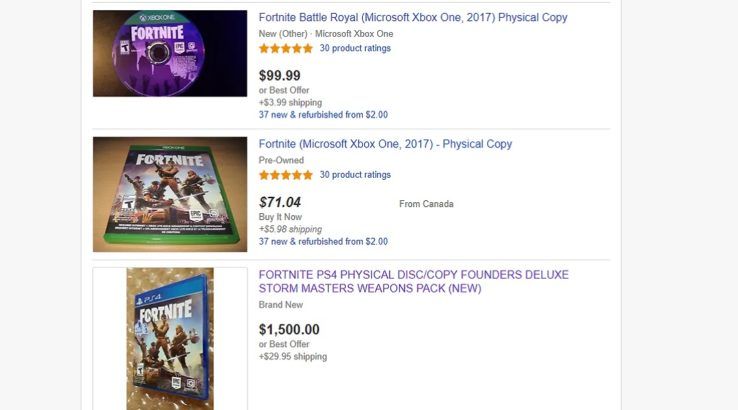This image features three rectangular boxes, each illustrating a different listing for the popular video game Fortnite, available on various platforms. Here are the detailed descriptions:

1. **Fortnite for Microsoft Xbox One (2017)**:
   - **Visuals**: The image includes a CD with the words "Fortnite" prominently displayed.
   - **Description**: It details "Fortnite Battle Royale" for Microsoft Xbox One, released in 2017.
   - **Condition**: The copy is new and comes in physical format.
   - **Price and Ratings**: Listed at $99.99 or best offer, with an additional $3.99 for shipping. It boasts a 35-star rating from 30 product reviews.
   - **Additional Info**: The listing mentions 37 new and refurbished copies available starting from $2, highlighted in blue.

2. **Fortnite for Microsoft Xbox One (2017) - Pre-owned**:
   - **Visuals**: Depicts the DVD cover of Fortnite for Xbox One.
   - **Description**: Includes specifics such as "Fortnite," alongside the release year (2017) and platform (Microsoft Xbox One).
   - **Condition**: This is a pre-owned physical copy.
   - **Price and Ratings**: Priced at $71.04 with a 5-star rating derived from 30 product reviews. Shipping costs $5.98 from Canada.
   - **Additional Info**: Similar to the first box, it mentions 37 new and refurbished copies from $2, in black text, with "Buy it now" displayed in gray text.

3. **Fortnite for PlayStation 4**:
   - **Visuals**: Displays the cover of the Fortnite PS4 version.
   - **Description**: This is a physical disc/copy referred to as the "Founder's Deluxe" edition, including the "Storm Masters" weapons pack.
   - **Condition**: New and brand new.
   - **Price and Offer**: Listed at a premium price of $1,500 or best offer.

This detailed depiction provides a thorough look into different listings for Fortnite across various gaming platforms, showcasing varying conditions and prices.